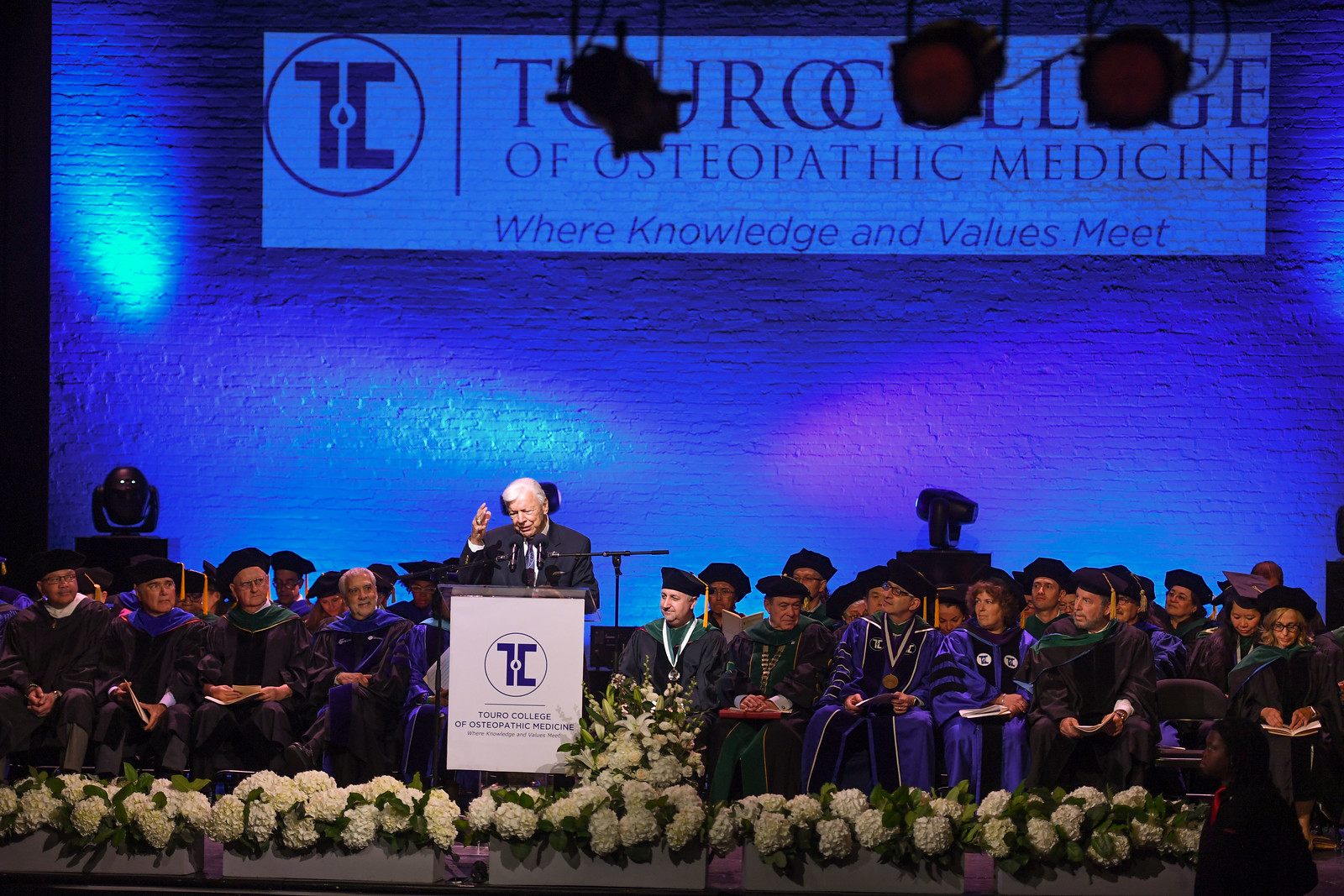In this wide rectangular image of a graduation ceremony, an elderly man with white hair stands at a white podium slightly to the left of the center. The podium reads "Turo College of Osteopathic Medicine" in purple. The man is wearing a suit and has one hand raised in the air, which features a prominent big ring. He addresses the audience through two microphones. Surrounding the base of the stage are several wide, gray rectangular boxes filled with thick white flowers. Behind the podium are a couple of rows filled with older men and women, donned in purple, gold, and green gowns along with black graduation caps. The backdrop is a brick wall illuminated to appear blue, and above it is a large white sign reading "Turo College of Osteopathic Medicine" and "Where Knowledge and Values Meet." In front of this sign, three large spotlights are positioned. The scene captures a moment of profound importance and celebration, encapsulated by the dignity and decorum of the occasion.